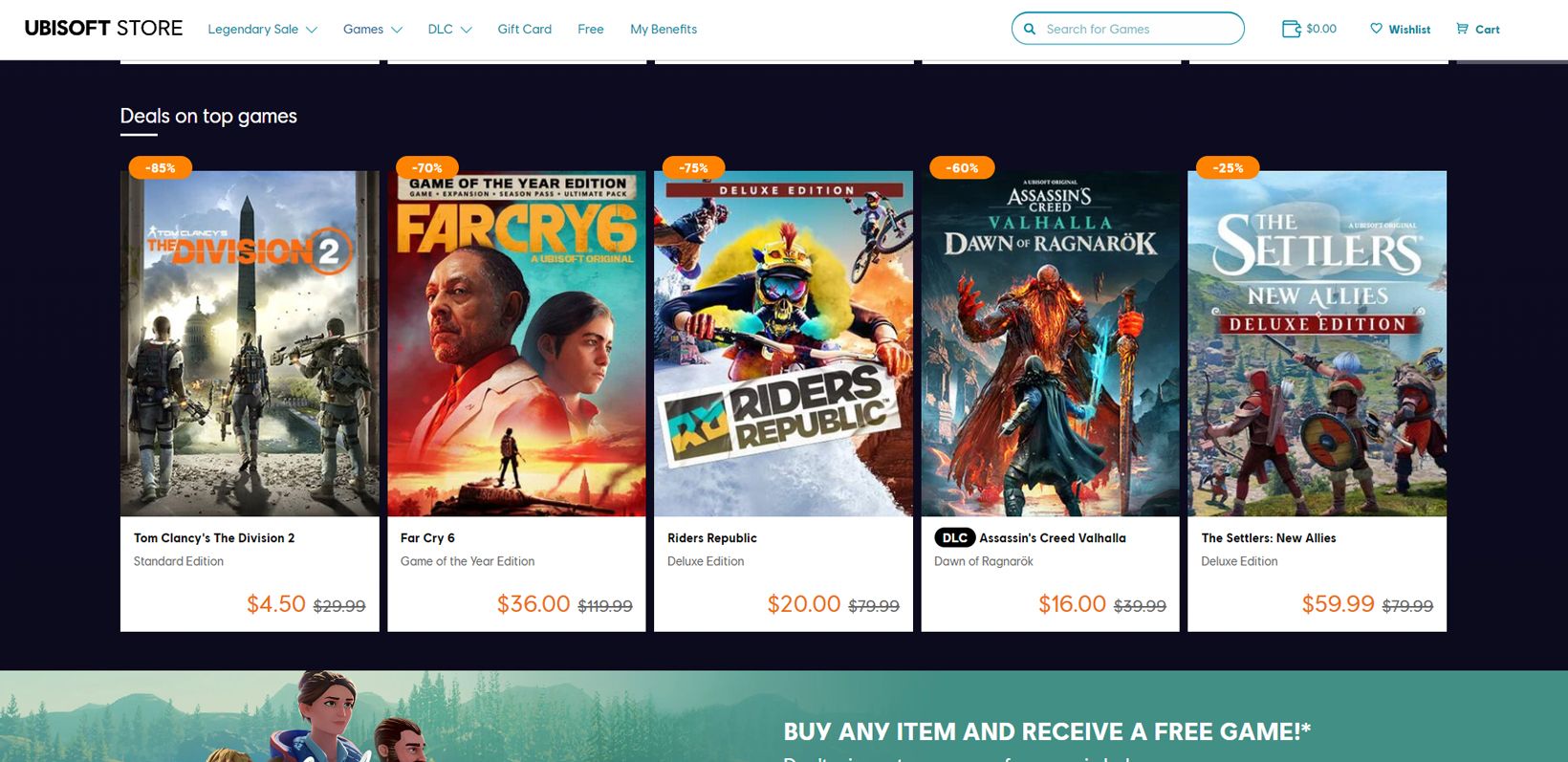The image features the Ubisoft Store webpage. At the top left, the Ubisoft logo and store name are prominently displayed. Next to them are small blue navigation menus labeled 'Legendary Sale,' 'Games,' 'DLC,' 'Gift Card,' 'Free,' and 'My Benefits,' each expandable to reveal more options. On the right side, there is a search bar, along with icons for viewing your cart, wishlist, and account credits.

Beneath this top section, a dark blue panel showcases tiles of popular games currently on sale. Among the highlighted deals are:
- **Tom Clancy's The Division 2 Standard Edition**, now priced at $4.50, down from $29.99.
- **Far Cry 6**, reduced to $36 from its original price of $199.99.
- **Riders Republic**, discounted to $20.
- **Assassin's Creed Valhalla**, now available for $16.
- **The Settlers: New Allies**, priced at $59.99.

At the bottom of the screen, a promotional green banner states: "Buy any item and receive a free game."

This detailed layout provides a clear and comprehensive overview of the Ubisoft Store's current offerings and promotions.